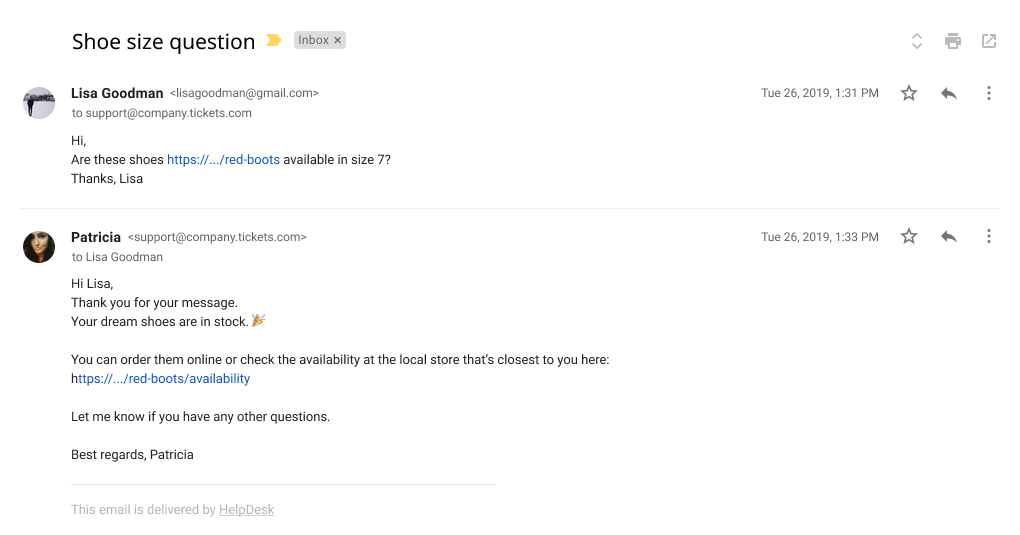A detailed descriptive caption for the image would be:

The image depicts an email exchange with a white background and black text. At the top, there is the Gmail interface including the inbox section, wherein a yellow arrow points towards it. There are two primary emails shown in this exchange.

The first email is from Lisa Goodman, sent on the 26th of a month in 2019 at 1:31 PM. Lisa's email address is displayed as lisagoodman@gmail.com, and her message is directed to support@companytickets.com. In her email, Lisa inquires about the availability of red boots in size 7 and includes a hyperlink: "https://redbootsavailableinsize7.com". The email is denoted with a star, an arrow, and three dots, which are part of the interface options.

The second email is a reply from Patricia, who represents the support team at companytickets.com. Patricia's response, timestamped at 1:33 PM on the same day, reassures Lisa that the red boots are in stock, advising her to either order them online or check the availability at the nearest local store using the link: "https://redbootsavailability.com". Patricia signs off by wishing Lisa well and offering further assistance. The email closes with a note that it was delivered by the helpdesk system.

Next to each email entry are small, indistinct profile pictures. Lisa's profile appears to be a landscape image of a person standing, while Patricia's profile is an image of a woman, though the details are hard to make out.